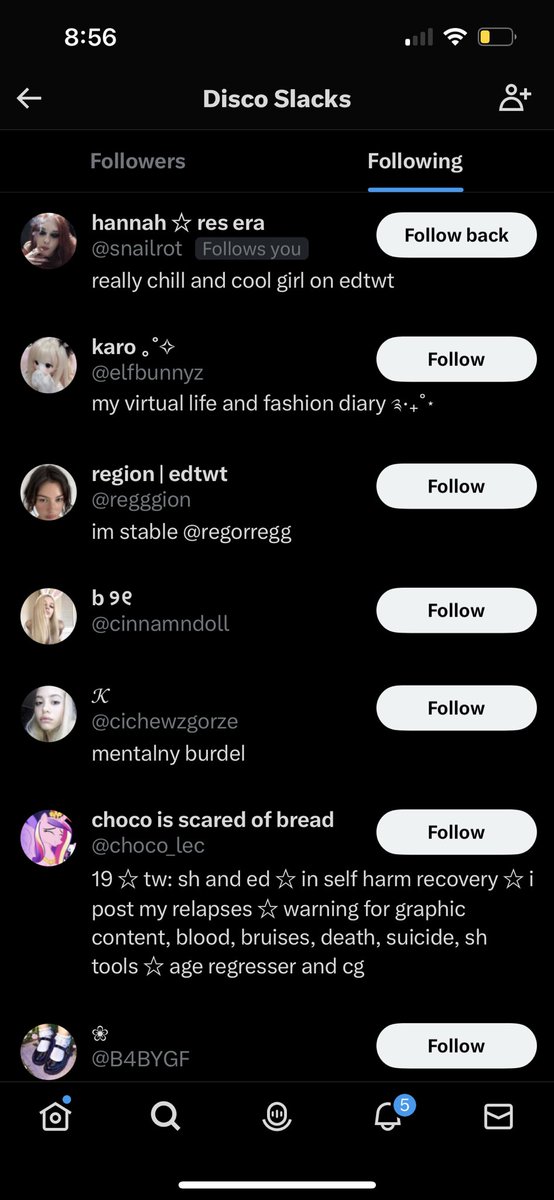**Screenshot Description: Detailed Overview of a Social Media Interface**

The image is a screenshot featuring a black background with predominantly white text. At the very top of the screenshot, the number "856" is displayed alongside a Wi-Fi icon, showing a single signal strength bar. A battery icon, indicating a yellow battery level, is also visible.

Beneath this, the primary content begins with the username "Disco Slacks" in white text at the top, accompanied by a white arrow. There is a small cartoon person icon with a plus sign next to it. Below this, there is a box with two tabs labeled "Followers" and "Following," with the "Following" tab underlined in blue, indicating it is the active tab.

The main section of the screenshot lists several usernames and their accompanying profile pictures, which are circular. Each entry also includes a white box with either "Follow Back" or "Follow" written inside:

1. **First User:**
   - **Username:** Hannah Ress Era
   - **Handle:** @SnailRot
   - **Bio:** "Follows You, Really Chill and Cool Girl on EDTWT, Follow Back"
   - **Action Box:** "Follow Back"

2. **Second User:**
   - **Username:** Caro
   - **Handle:** @ElfsBunnies
   - **Bio:** "My Virtual Life and Fashion Diary, Region EDTWT at Region I'm Stable at ReGoreGG, B9E at Cinnamon Doll"
   - **Action Box:** "Follow"

3. **Third User:**
   - **Username:** K
   - **Handle:** @SeechGores
   - **Bio:** "Motholony Burr Doll, Choco is Scared of Bread"
   - **Action Box:** "Follow"

4. **Fourth User:**
   - **Username:** 19 Star
   - **Handle:** @Choco_LEC
   - **Bio:** "Trigger Warning, SH and ED and Self Harm Recovery. I Post My Relapses, Warning for Graphic Content, Blood Bruises, Death, Suicide, SH Tools, Age Regressor and CG."
   - **Action Box:** "Follow"

5. **Fifth User:**
   - **Username:** B4BYGF
   - **Handle:** Not specified
   - **No Bio Provided**
   - **Action Box:** "Follow"

At the bottom of the screenshot, there are several icons in white, including a house, a magnifying glass, a microphone, a bell with a blue circle and the number five, and an envelope. A thin white line borders the bottom of the interface.